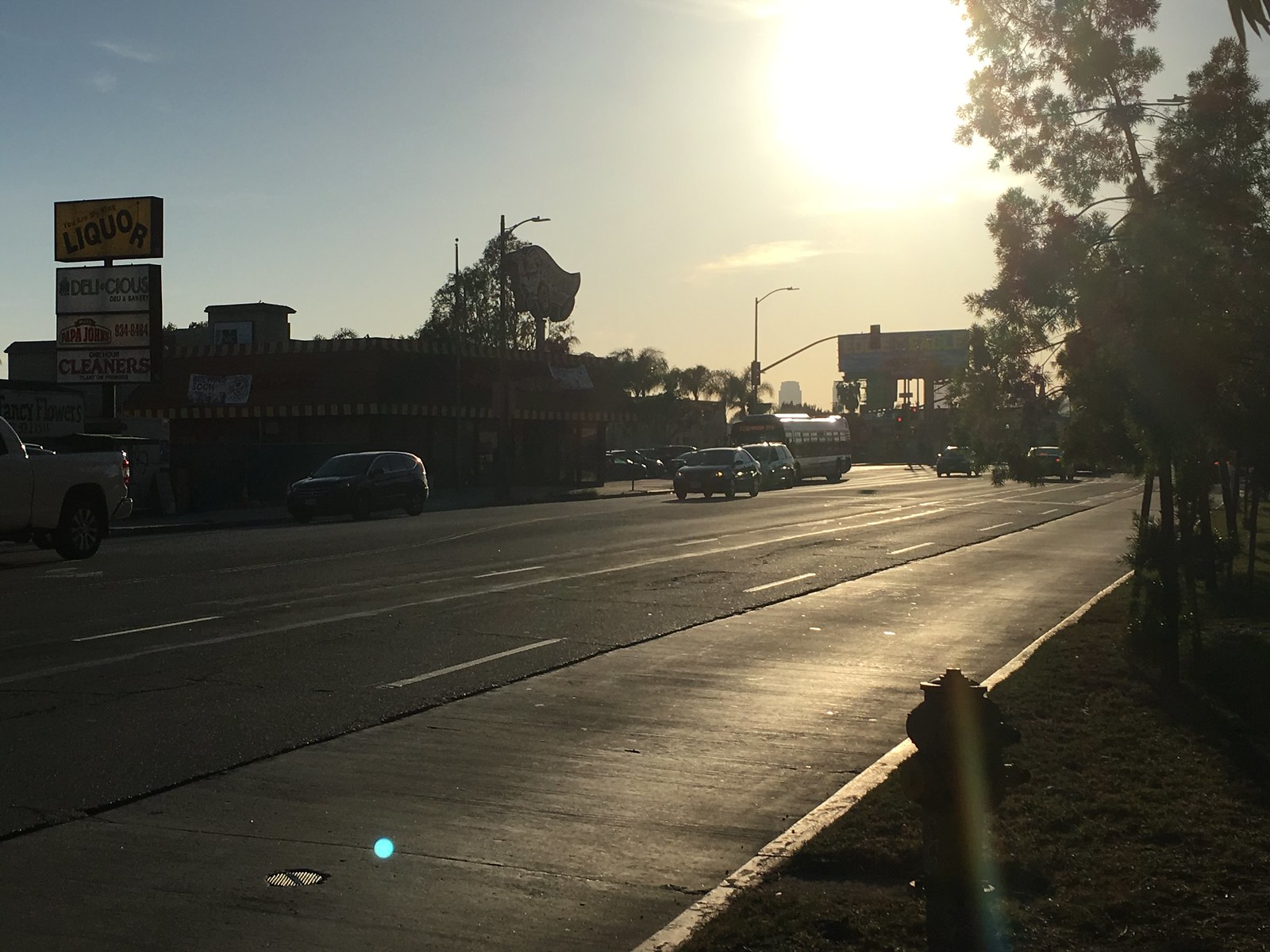This photograph captures a sunny day on a bustling road. Multiple cars and a bus are visible, traveling past a strip mall in the background. The sun is prominent in the sky, casting a lens flare that includes a noticeable green dot and sunbeam rays, partially obstructing the view of a fire hydrant. Stoplights and a light pole are present amidst the scene, while trees with leaves and patches of grass add a touch of greenery. The road features white lane markings. The strip mall's signage indicates several businesses: a liquor store with yellow and black lettering, a deli with white text on a dark font, a Papa John's with a white background, and a cleaners business below it. Additionally, a banner hangs on one of the buildings, contributing to the lively atmosphere of this suburban setting.